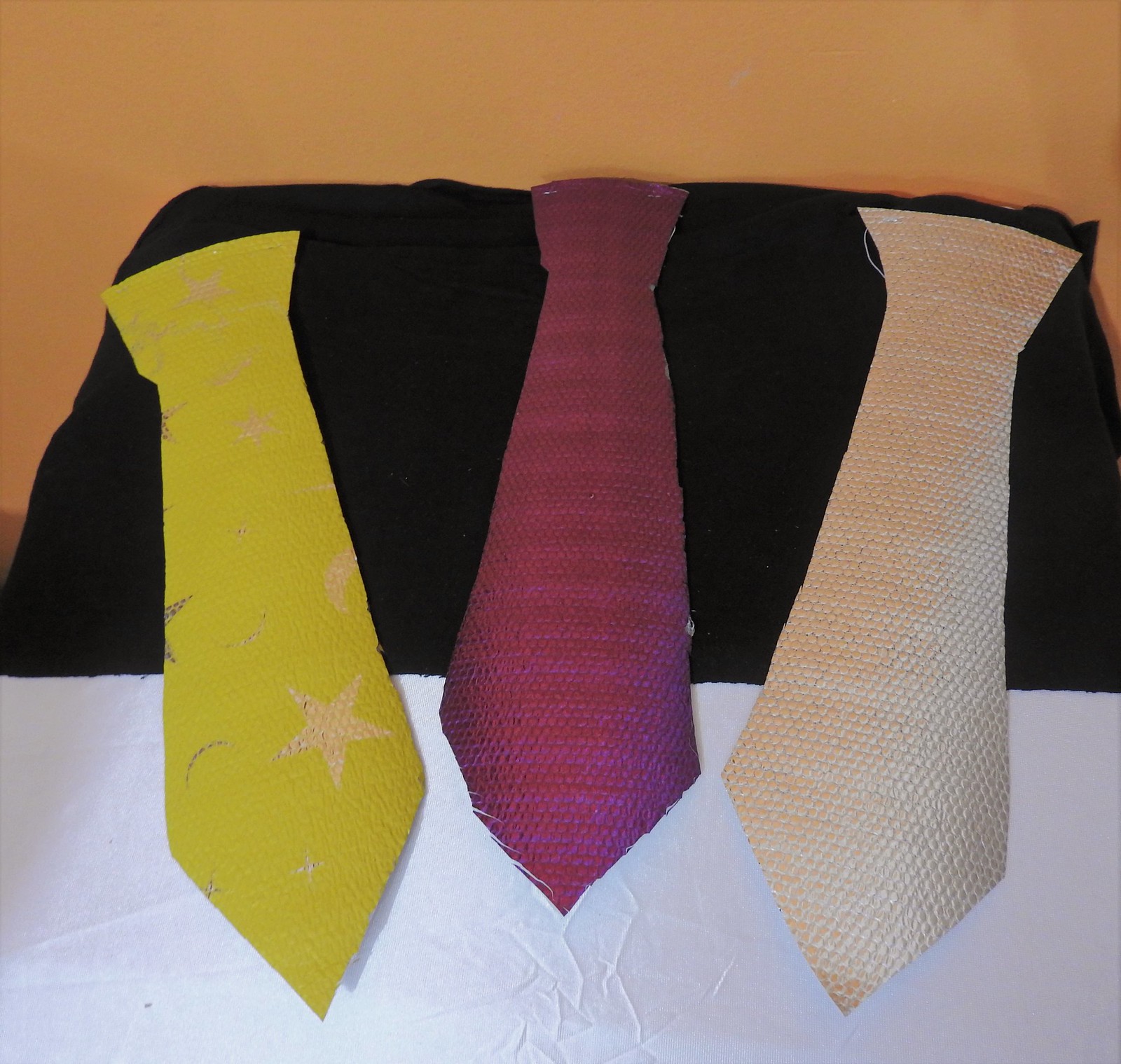The photograph showcases three uniquely crafted ties, each made from textured materials rather than traditional fabric. Positioned against a multi-layered background, the image features an orange upper section and a lower part that's divided into a black and white fabric. The left tie boasts a vibrant yellow color adorned with gold moons and stars, reminiscent of traditional star illustrations. The middle tie, a striking purple with a slightly metallic sheen, offers a bold contrast. The right tie features a subtle snakeskin-like texture, rendered in a muted silverish-gold hue. All three ties exhibit rough, handmade edges, adding to their distinct charm.